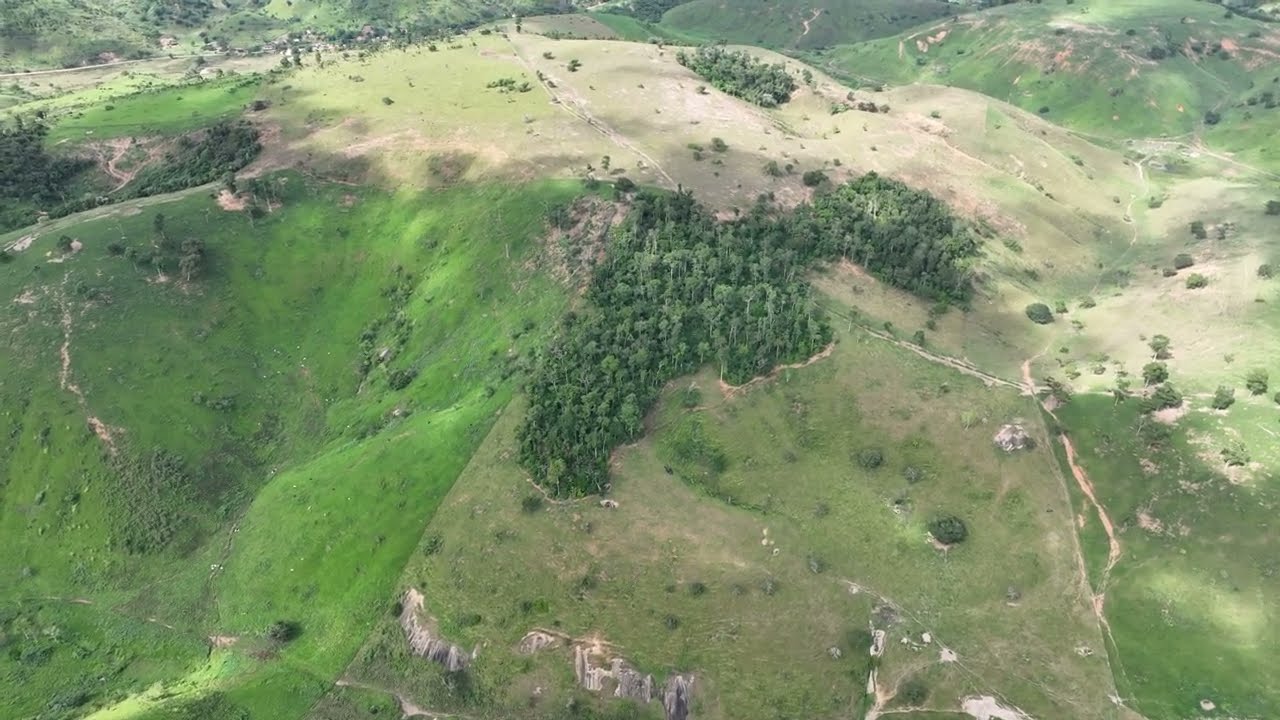The image is an aerial photograph showcasing a hilly landscape with distinct peaks and valleys. At the center of the photo, there is a prominent, isolated grouping of darker green trees, forming a small forest-like island amidst the otherwise sparse vegetation. Another cluster of trees is visible towards the upper back part of the image, adding depth to the scene. Sporadic trees dot the landscape, but the majority of the area appears barren, with green grass patches primarily on the left side. This grassy area transitions into a dipped valley, providing a rich, verdant contrast to the surrounding hilly terrain, which features varying tones of green and brown dirt. Trails or roads can be seen meandering through the hills, adding a sense of scale and direction to the photograph. The hills showcase a mixture of elevations, with the higher parts towards the center right and upper left and valleys and dips along the bottom left and back side, creating a dynamic and diverse topography.